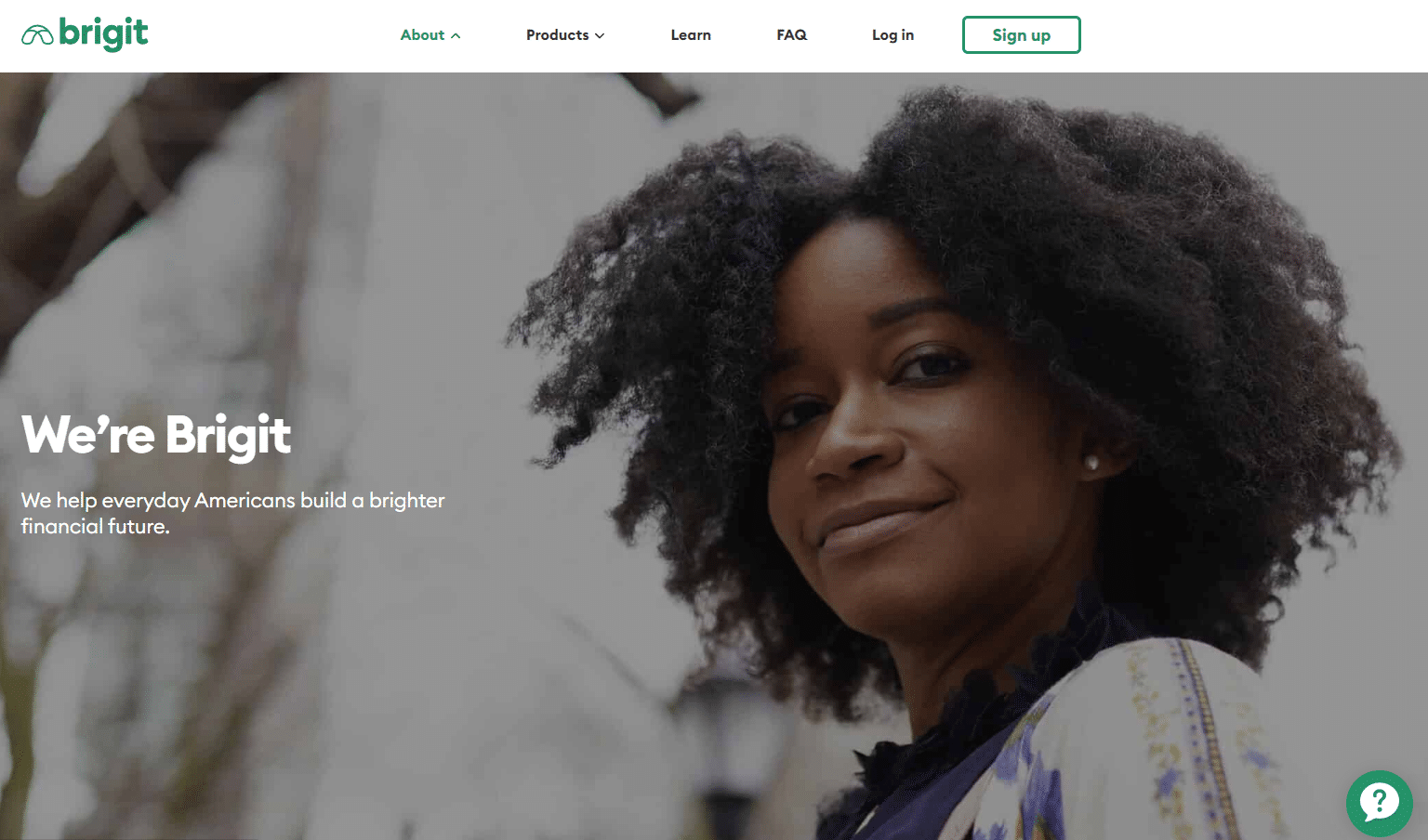Screenshot of the Bridget website showcasing an African American woman smiling with short, thick hair and brown eyes, adorned with an earring. She is wearing a purple and white shirt with ruffles along the neckline. The website features a green Google logo and a navigational bar with tabs for 'About,' 'Products,' 'Learn,' 'FAQ,' 'Login,' and a green 'Sign Up' button. To the left of the woman, white text reads, “We’re Bridget. We help everyday Americans build a brighter financial future.” A tree image decorates the background, and a question mark is visible in the corner.